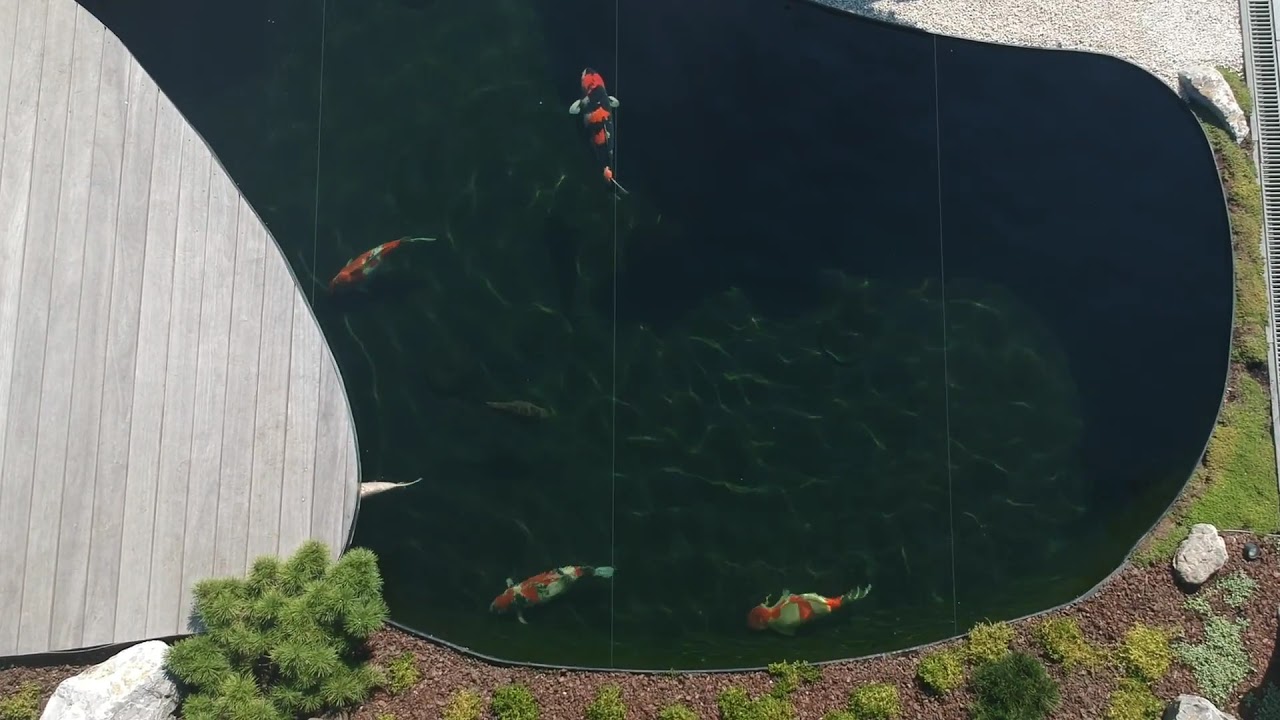In this overhead shot, a backyard koi pond is framed by earthy tones of dirt and bark, interspersed with patches of grass, little bushes, trees, and scattered rocks. The water in the pond appears almost black due to its depth, providing a striking contrast to the vibrant koi fish swimming within. We can see four, possibly five koi fish, each displaying a variety of colors – black, red, gray, orange, and white. One fish at the far left stands out for being entirely white. The largest koi, with an appearance suggesting a piranha, swims among others with mottled and striped patterns. The pond itself is irregularly shaped, occupying around 60% of the visible area of the image. On the left side, a light gray wooden deck extends slightly over the water, offering a viewing platform. The edges of the pond are lined, suggesting clear boundaries for the water, with additional lining visible at the top right of the image. This serene depiction may have been captured from a drone or a raised deck, showcasing the calm, reflective water surface and the lively, colorful fish in their tranquil habitat.